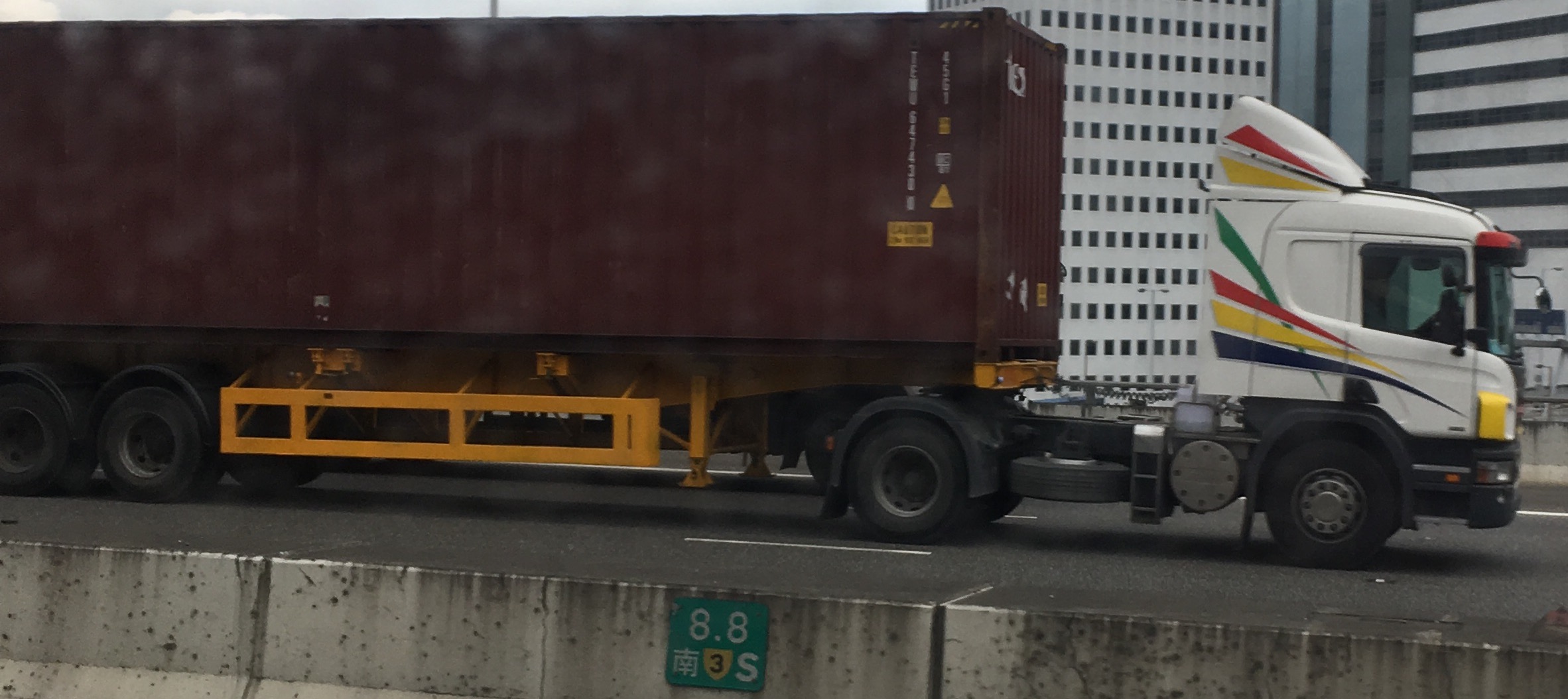The image showcases a white semi-truck with an 80s-style design featuring green, red, yellow, and navy stripes driving down a road, possibly on a bridge. The truck is hauling a burgundy-brown container with white writing and yellow labels, loaded with numerous black tires. The truck's cab has windows, and a driver can be seen inside. There's an orange undercarriage visible beneath the truck. In the background, tall white buildings with many small windows and a grayish-blue office building are seen. A green sign near the truck displays "8x8" along with Chinese symbols and the number "3S," suggesting an Asian locale. The road has a gray, dirty divider marked by black mildew and dirt.